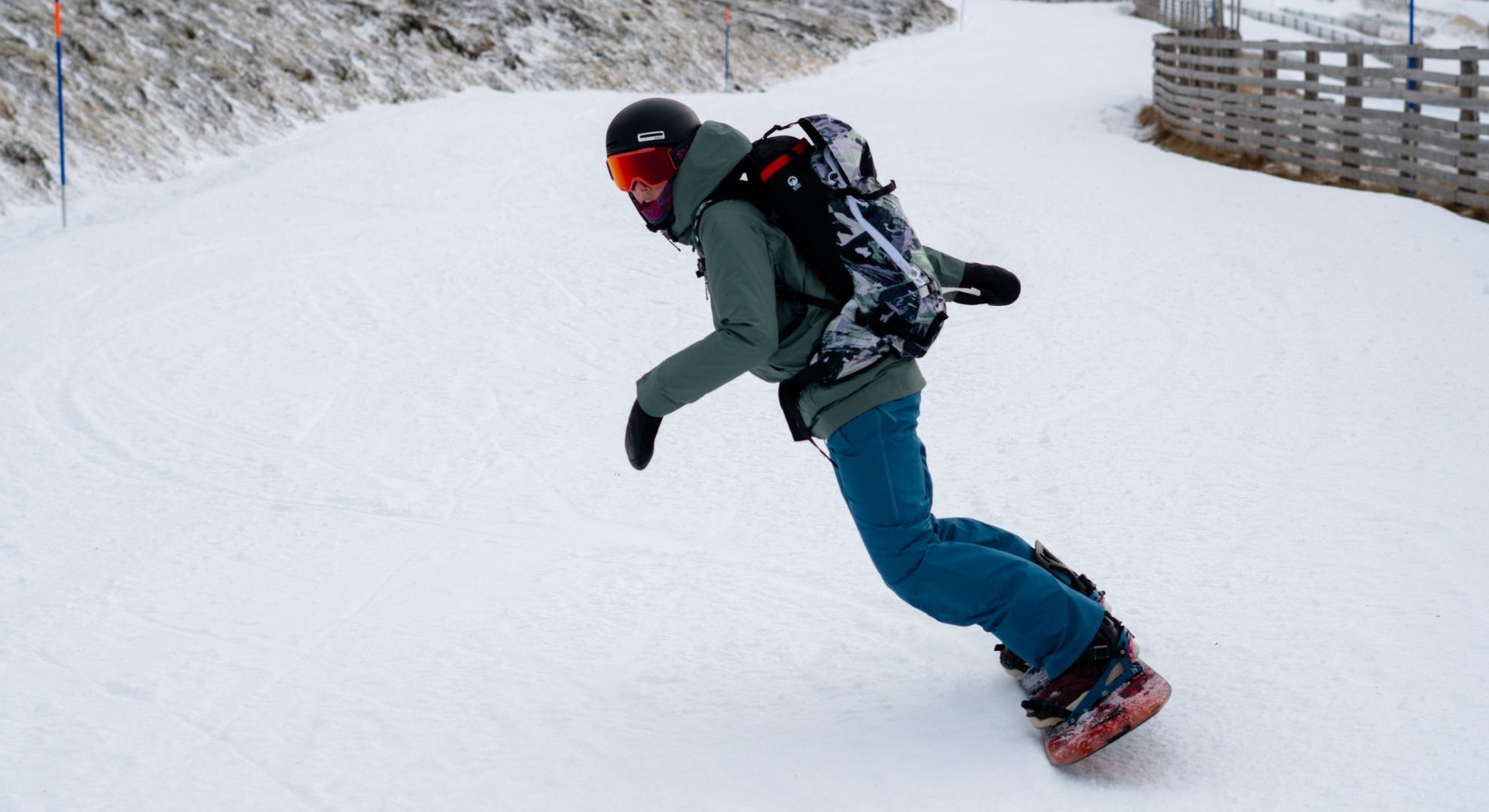This vibrant color photograph captures a dynamic scene of a snowboarder gliding across a snow-covered path, leaning forward at almost a 45-degree angle. The image showcases the snowboarder dressed in a distinctive ensemble: a green jacket, denim pants, black gloves, red snow goggles, and a black helmet. They carry a black and white patterned backpack and are secured to a red snowboard. The landscape features a wooden fence curving along the right side of the path, while the left side displays a rocky texture indicative of a hillside. The tracks left behind by the snowboarder are clearly visible, and there are markers along the path. The setting is serene with no other people, animals, or birds in sight. The path is part of a larger snowy terrain with additional trails visible in the background, enhancing the sense of adventure in this solitary snowboarding journey.